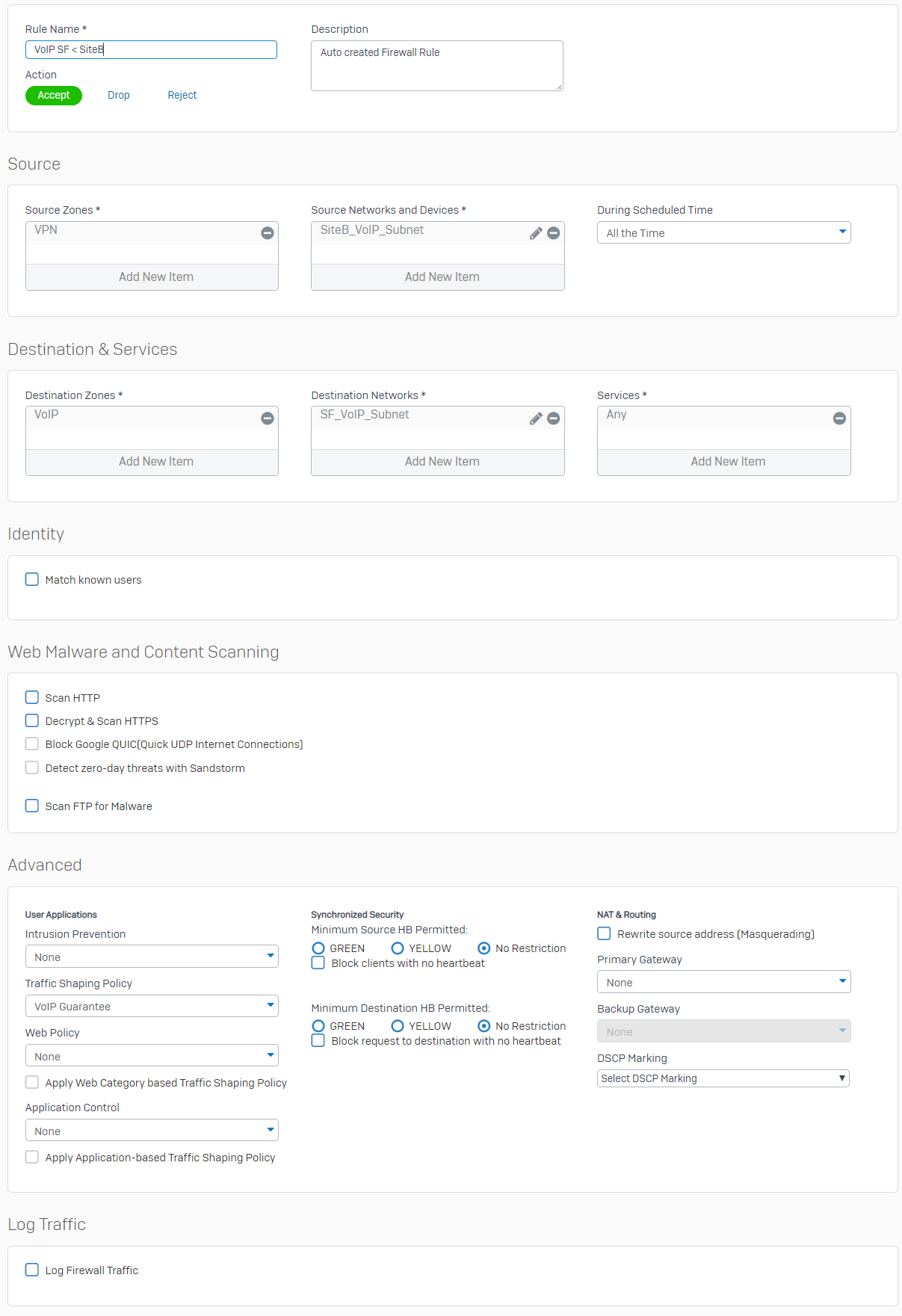**Caption:**

The image displays an interface screen for network security and firewall configuration. In the top-left corner, there is a field labeled "Role Name" associated with the designation "DOIP," indicating it's a Site P. Below this, an auto-generated description details the firewall's setup. 

The interface allows actions such as "Accept," "Drop," or "Reject" for various network parameters. Key sections of the interface include:

- **Source:** 
  - Source Zone
  - VPN
  - "Add New Item" button
  - Source Network, representing Site P (DOIP) Subnet, with options to edit (pencil icon), or remove (minus icon)
  - Scheduling options: "During Scheduled Time" or "All the Time"

- **Destination Services:**
  - Destination Zone
  - Star (indicative of any/all matches)
  - DOIP, with edit and remove options
  - Destination Networks labeled "SF_DOIP_Subnet"
  - Services: Star (any), with options to add, remove, and edit services

- **Identity:**
  - A checkbox for matching known users, currently unchecked
  - A white box containing text "Web Malware and Content Scanning"

Within the "Web Malware and Content Scanning" section, there are checkboxes for:
  - "Scan HTTP"
  - "Decrypt and Scan HTTPS"
  - "Block Google"
  - Text mentioning "qic" and a code "10x0d3"
  - "Scan HTTP for Malware"
  - "Advance Disinformation"

Additionally, there are options under "Lock Traffic":
  - The checkbox "Lock Firewall Traffic" is currently unchecked.
  - Options related to "Unrooting."

The overall interface supports comprehensive customization for firewall rules, network traffic management, and security scanning settings.